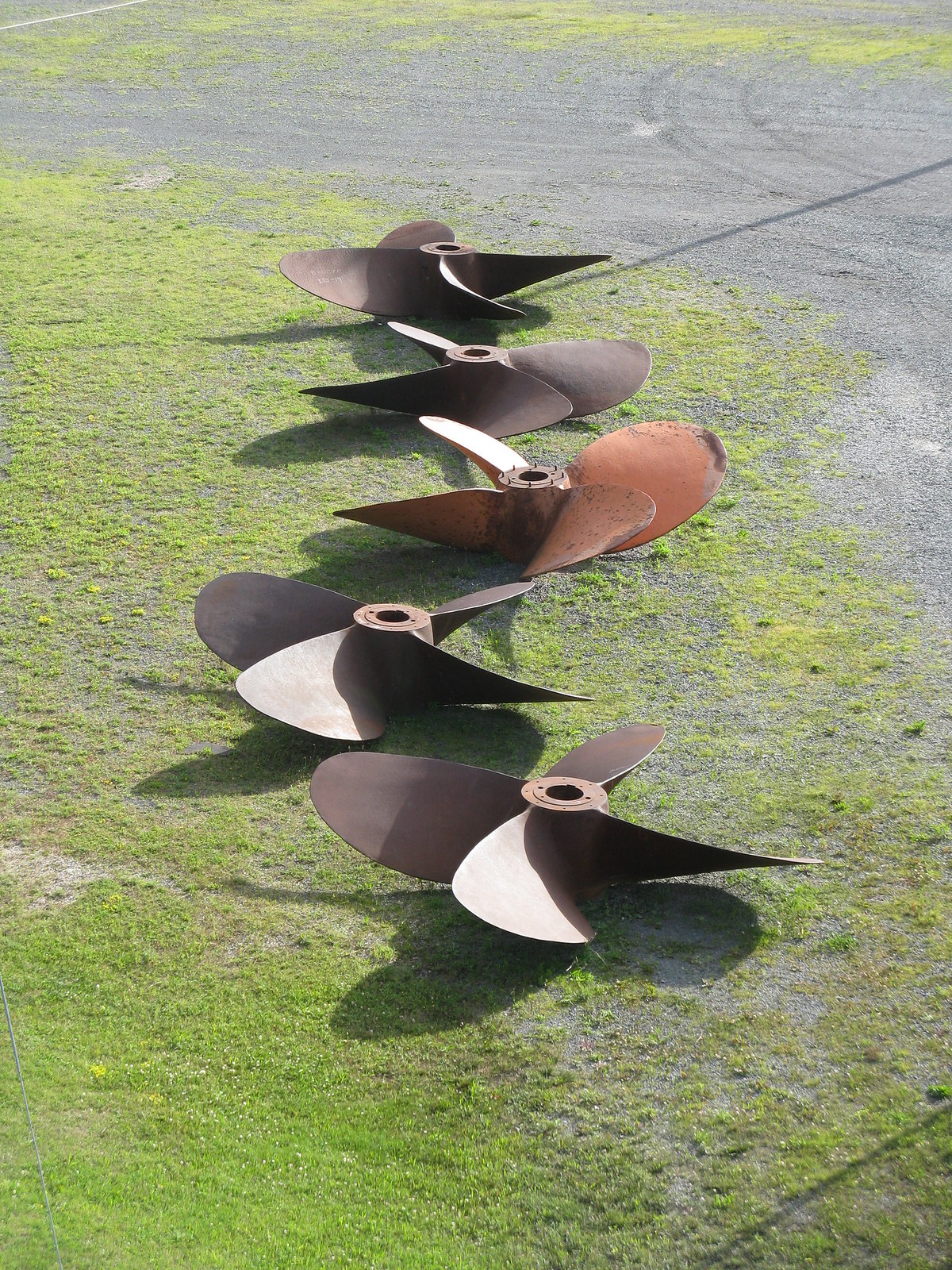The image features a row of five boat propellers positioned on a light, sparse grass field. The grass is interspersed with a few stones and there's a distinct, grassless path indicating a drive or motor path nearby. The propellers are aligned horizontally from the camera's perspective, stretching front to back. The central propeller stands out with its badly rusted and bronze appearance, suggesting significant wear, while the surrounding four propellers exhibit a newer, grayish hue. Each propeller consists of bent blades joined in the center by a circular hub, and shadows are cast on both the top and bottom right edges of the scene.